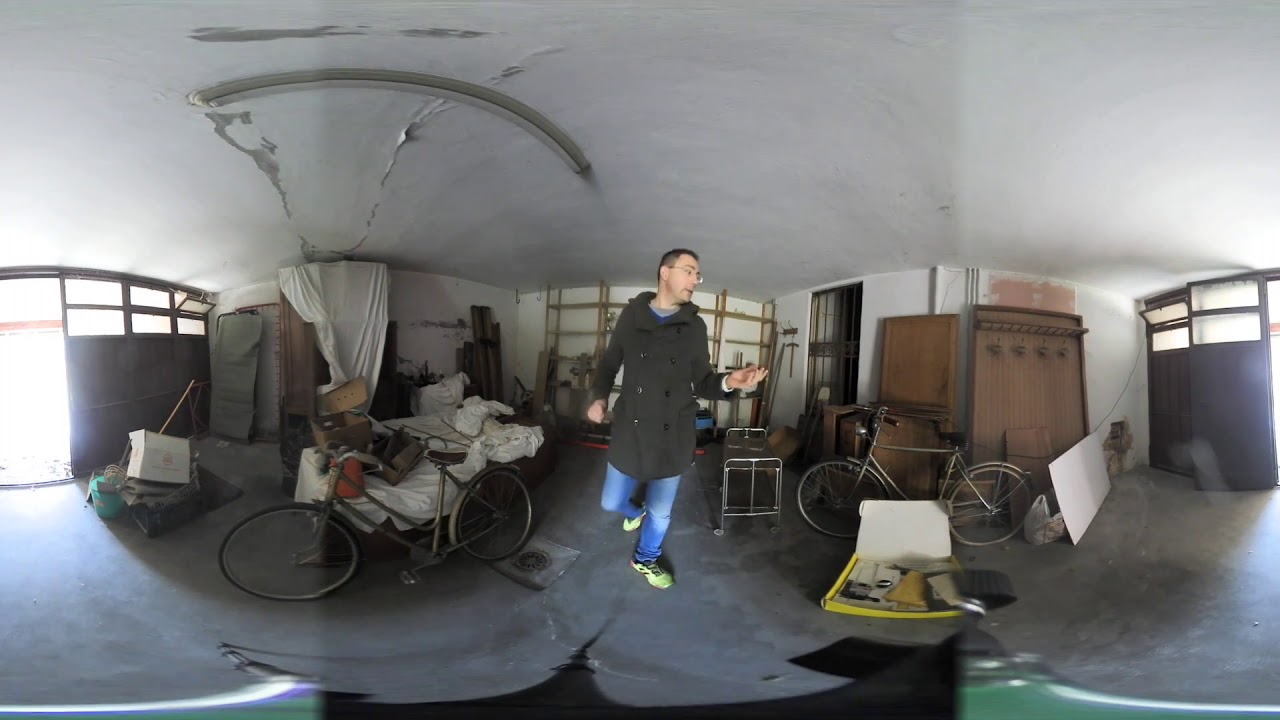In this panoramic image of a garage-like interior, the viewer's perspective is stretched to show all the walls in a distorted fashion, causing the angles where the walls meet the ceiling to curve upward. The setting is cluttered with various items, including several bicycles and disorganized furniture covered with rags and bedsheets. To the left, an open sliding door provides a glimpse outside. 

Centered in the image stands a white male with glasses, donning a black trench coat that features prominent buttons, jeans, and green cross-trainer shoes with yellow accents. He is positioned between two bicycles, one of which is silver with a green triangle-shaped frame visible at the bottom middle of the image. The garage walls are a mix of eggshell white and other shades, complemented by dark brown shelving and doors. The ceiling and floor present in light gray hues.